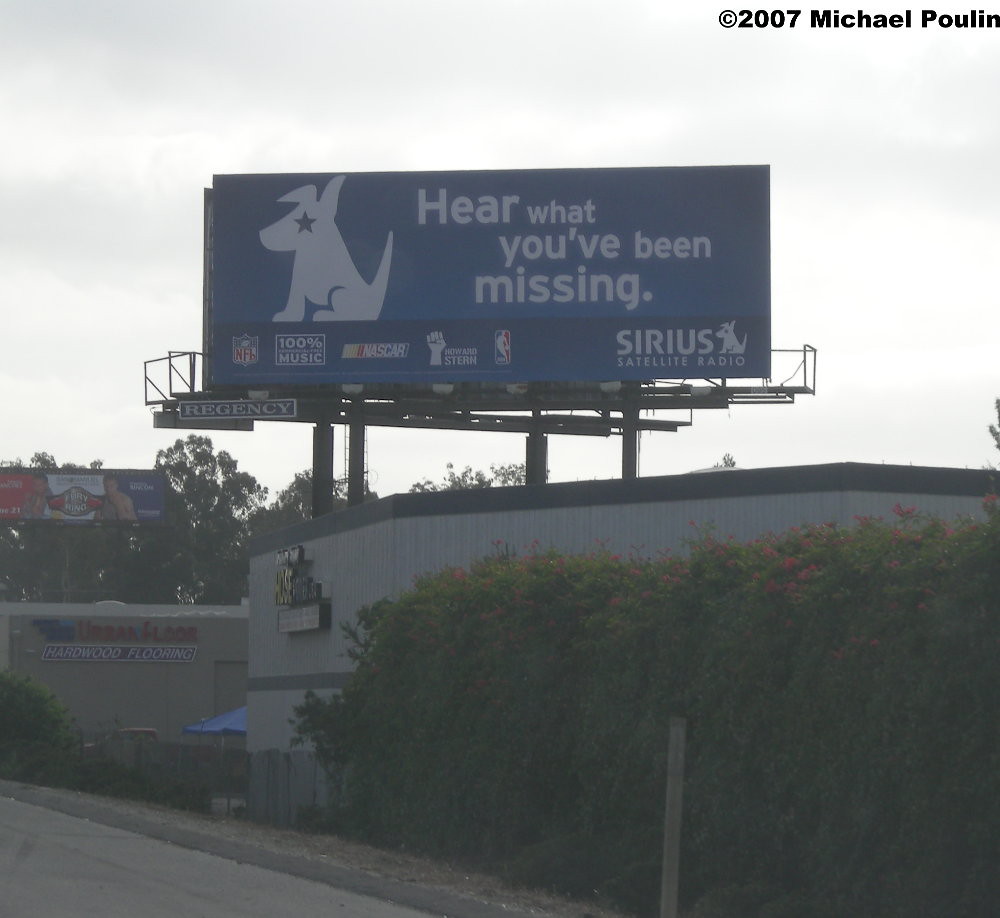The picture captures a detailed scene of a cloudy day with a gray, overcast sky. Centered prominently is a large, eye-catching billboard with a dark navy blue background, perched on black posts and sporting a black frame. The billboard's text reads in bold white letters, "Hear What You've Been Missing," and promotes Sirius Satellite Radio. A striking graphical image of a white dog with a blue star for an eye grabs attention on the left, while an array of logos for popular entertainment sources including the NFL, NASCAR, Howard Stern, NBA, and "100% Music" highlight the variety offered by the service.

In the bottom corners, the billboard repeats "Sirius Satellite Radio" with another dog logo beside it. In the top right corner is a copyright notice: "© 2007 Michael Poulin," with the M and P capitalized. Below the billboard, a smaller sign reads "Regency," located on the bottom left. 

The background features an assortment of buildings, including a tan and gray structure with a sign for "Hardwood Flooring," though the full name isn't visible. To the left of the main billboard, part of another red, white, and blue billboard peeks into view, potentially promoting WWE wrestling as it depicts championship belts and figures. The scene is completed with green shrubs, bushes, and a smattering of trees scattered throughout the background, alongside a partly visible road running by the billboards and buildings.